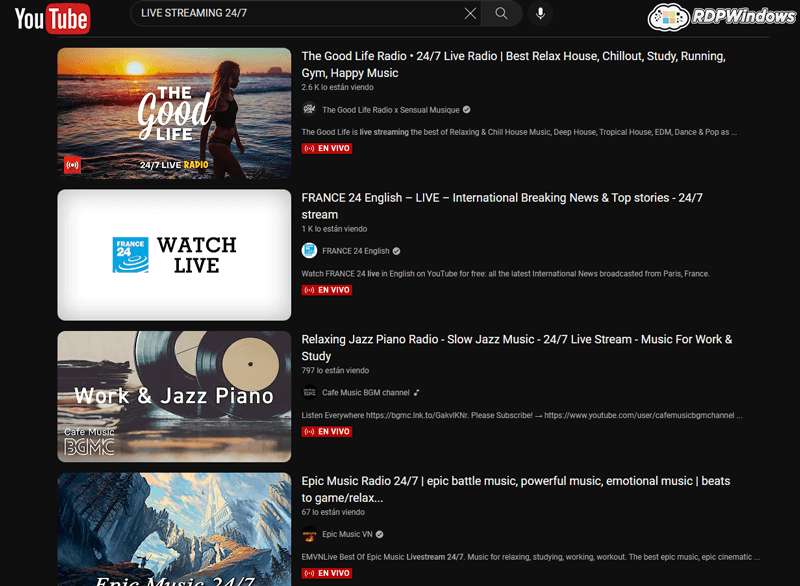This is a detailed caption for an image that is a screenshot of YouTube in dark mode. The background of the interface is black, creating a stark contrast for the elements shown. In the upper left corner, the YouTube logo is prominently displayed. The logo features the word "You" in white font followed by "Tube" also in white font, but the latter is enclosed within a red rectangle with rounded edges. Adjacent to the logo on the right is a search bar, in which the user has typed "live streaming 24-7." At the end of the search field are three icons: a small 'X' for clearing the search text, a magnifying glass for initiating the search, and a microphone for voice search.

In the extreme upper right corner of the screenshot, a watermark indicating the hosting platform is visible, reading "RDP Windows." Directly below this, the main content of the YouTube page is visible, featuring four video thumbnails with accompanying information to the right. 

The first video entry at the top displays a thumbnail of a woman in a bikini walking along a beach during sunset, with the sky painted in warm hues. Superimposed in white text over the center of the thumbnail are the words "The Good Life." Below this thumbnail, the title is further detailed as "24-7 Live Radio." To the right side of the thumbnail, the channel information and video description follow: "The Good Life Radio. 24-7 Live Radio. Best Relaxed House Chill Out Study Running Gym Happy Music." This comprehensive description succinctly captures the essence of the channel as a source for continuous, relaxing house music suitable for various activities.